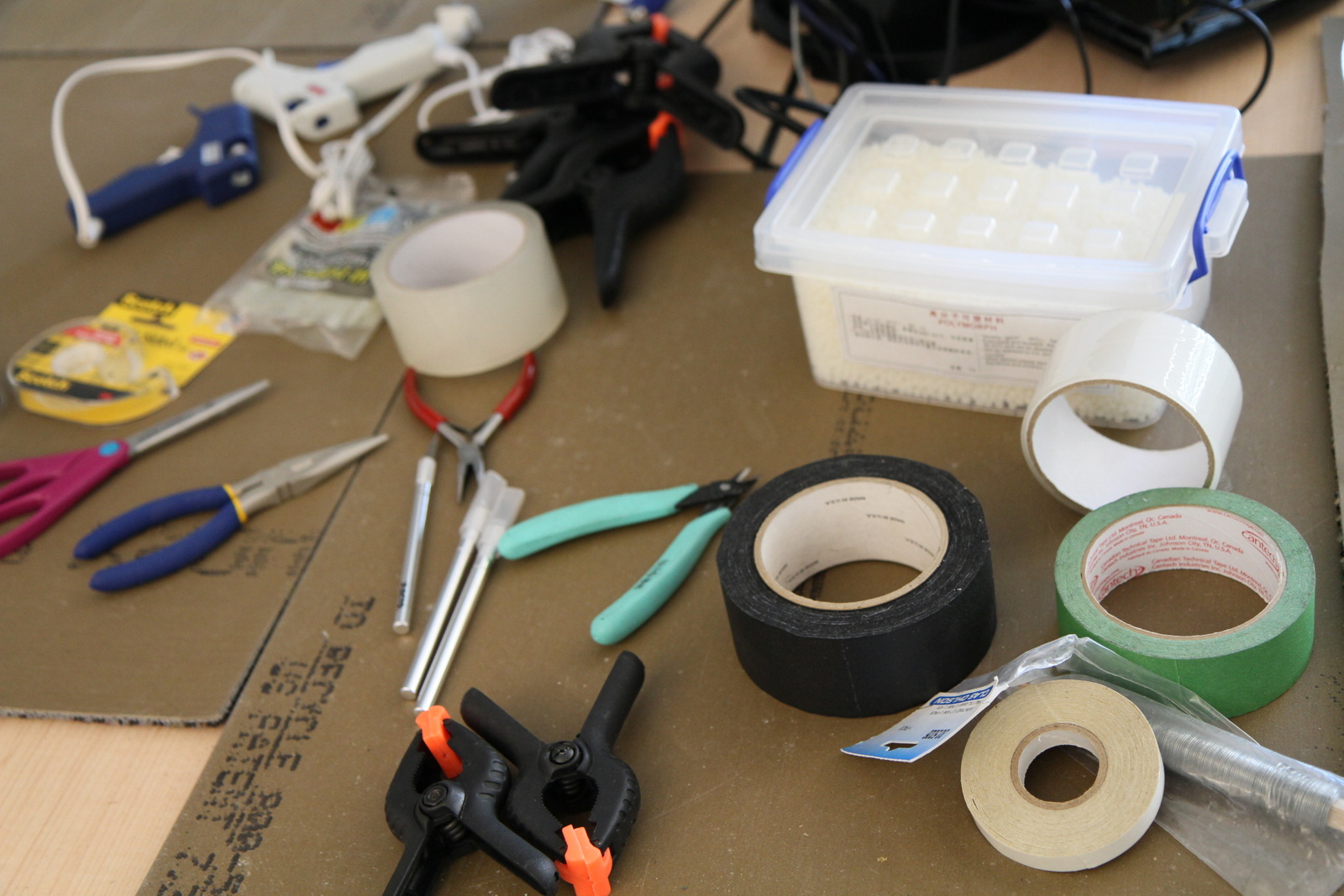Various tools and implements are scattered across a table, ready for different types of projects. The surface consists mainly of a darker brown mat, which appears to have a fabric edge underneath, contrasting with the light blonde-colored table that is visible in the bottom left and upper right corners of the image. The brown mat features some black writing, though it's not clearly legible.

On this mat, numerous items are arranged: several rolls of tape including white, green, and black masking tape along with clear packaging tape; a plastic container resembling a Q-tip holder; a spool of wire thread in a plastic bag; and black clamps with distinctive orange ends. There are various kinds of needle-nose pliers, a pair of scissors with maroon handles, a yellow package of Scotch tape, another roll of clear packaging tape, more black clamps with orange tips, and both a white and a blue hot glue gun. This eclectic assortment of tools appears ready to tackle an array of creative and maintenance tasks.